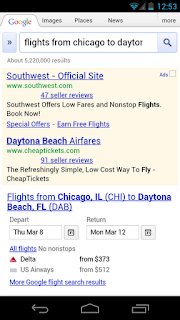This screenshot is of a webpage displayed on a cell phone. At the very top is a black status bar. The left side of the bar is empty, while the right side features an icon resembling a heart, along with indicators showing the battery is nearly depleted and the time is 12:53.

Just below the status bar is a section with navigation tabs labeled "Google," "Images," "Places," "News," and "More." The "Google" tab is selected, displaying Google's colorful logo. Beneath the logo is a search bar containing the query, "flights from Chicago to Dayton."

Below the search bar, it states there are about 5,220,000 results. The results begin with a highlighted section for ads. The first ad is from Southwest, labeled as the official site with 47 seller reviews, promoting low fares and non-stop flights, encouraging users to book now. It also mentions special offers for earning free flights. The second ad promotes Daytona Beach Airfares on www.cheaptickets.com, with 91 seller reviews. The ad describes it as a simple, low-cost way to book flights.

The main content background is white, presenting information about flights from Chicago, Illinois to Daytona Beach, Florida. It provides options to select departure and return dates. The results indicate there are no non-stop flights available, listing Delta with prices starting at $373 and US Airways from $512. At the bottom of the section, there is an option to view more Google flight search results.